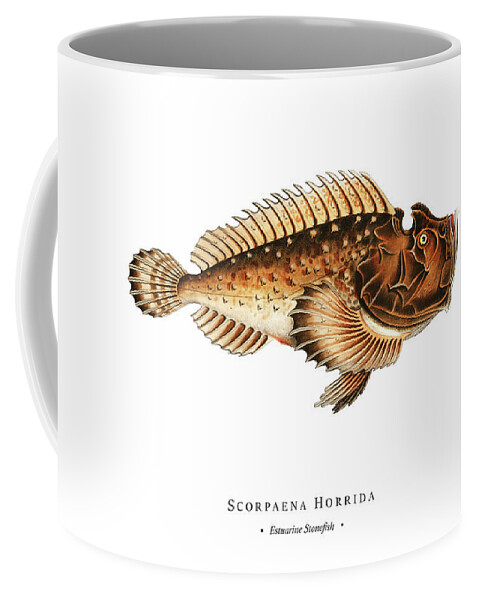The image depicts a bright white, shiny mug with a detailed design featuring a brown fish with distinctive fins, including a dorsal fin and spiny, fan-like fins. The fish illustration appears to be a scorpionfish, notable for its historical and somewhat intricate appearance, with a brown body and a white belly. At the bottom of the mug, there are black letters reading "Scorpaena horrida," indicating the scientific name of the estuarine stonefish. Below this, in much smaller, almost blurry text, it says "estuarine stonefish." The mug has a white handle and is set against a solid white background. The natural light enhances the clarity of the image, making all details easily visible.